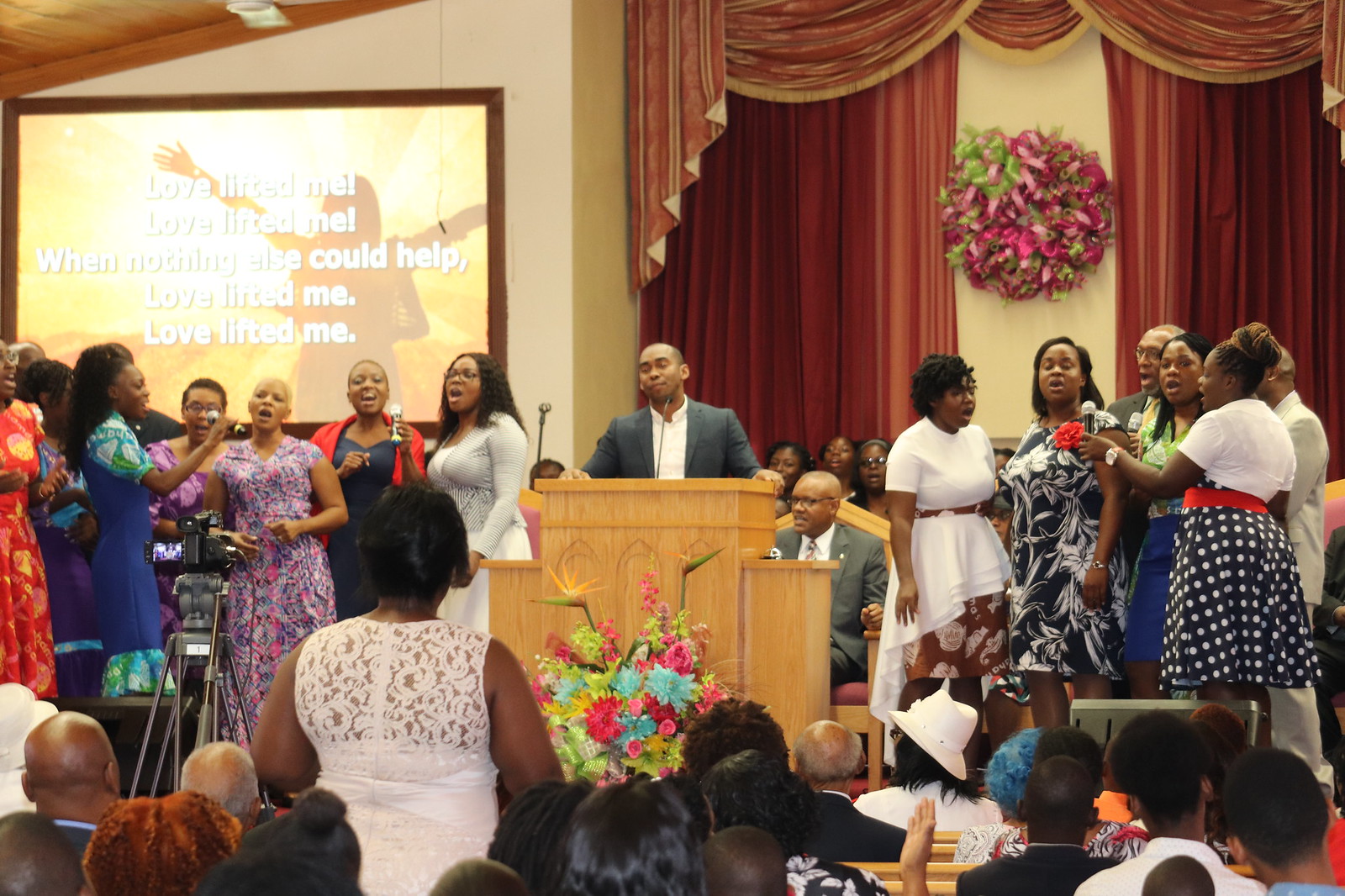Inside the bustling church, a dynamic scene unfolds. At the center, a black man stands behind a wooden-colored podium, gripping a brown microphone with both hands raised and eyes closed, clad in a gray jacket and a white shirt, leaning slightly left. In front of the podium, a vibrant bouquet featuring blue and pink flowers interspersed with green leaves adds a touch of natural beauty. To the left and right of him, groups of women form semi-circles around microphones, engaged in a choir performance. One distinguished singer on the far right holds a red flower, while dresses range from white, black and white patterns, to a striking black skirt with white dots. Above these singers, a large screen displays the lyrics "Love lifted me, love lifted me when nothing else could help, love lifted me," glowing with bright yellow light despite a slight glare affecting readability. Amber-colored curtains hang straight down at the back, flanked by a wreath adorned with purple and green hues. The congregation fills the pews, including a noticeable woman in a sleeveless white dress with lace standing amidst a sea of seated churchgoers, their attentions divided between the powerful sermon and the harmonious singing.